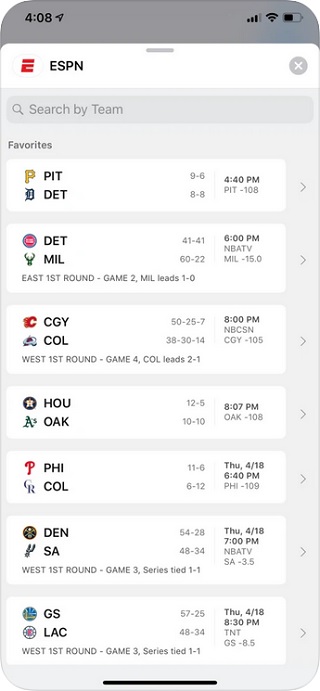The image showcases a mock-up of a phone screen displaying the ESPN app, which provides scores and schedules for various sports events. The top of the screen features the ESPN logo, accompanied by a search bar labeled "Search by team." The interface is populated with a list of favorite teams, indicated by their logos and names on the left side. 

The app displays a range of upcoming games across different sports, featuring matchups such as:
- Pittsburgh Pirates vs. Detroit Tigers (Baseball)
- Detroit Pistons vs. Milwaukee Bucks (Basketball)
- Calgary Flames vs. Colorado Avalanche (Hockey)
- Houston Astros vs. Oakland Athletics (Baseball)
- Philadelphia Phillies vs. Colorado Rockies (Baseball)
- Denver Nuggets vs. San Antonio Spurs (Basketball)
- Golden State Warriors vs. Los Angeles Clippers (Basketball)

The color scheme predominantly consists of light gray and white backgrounds, with black text for easy readability. Each sports entry is neatly organized, allowing users to quickly identify teams and upcoming games.